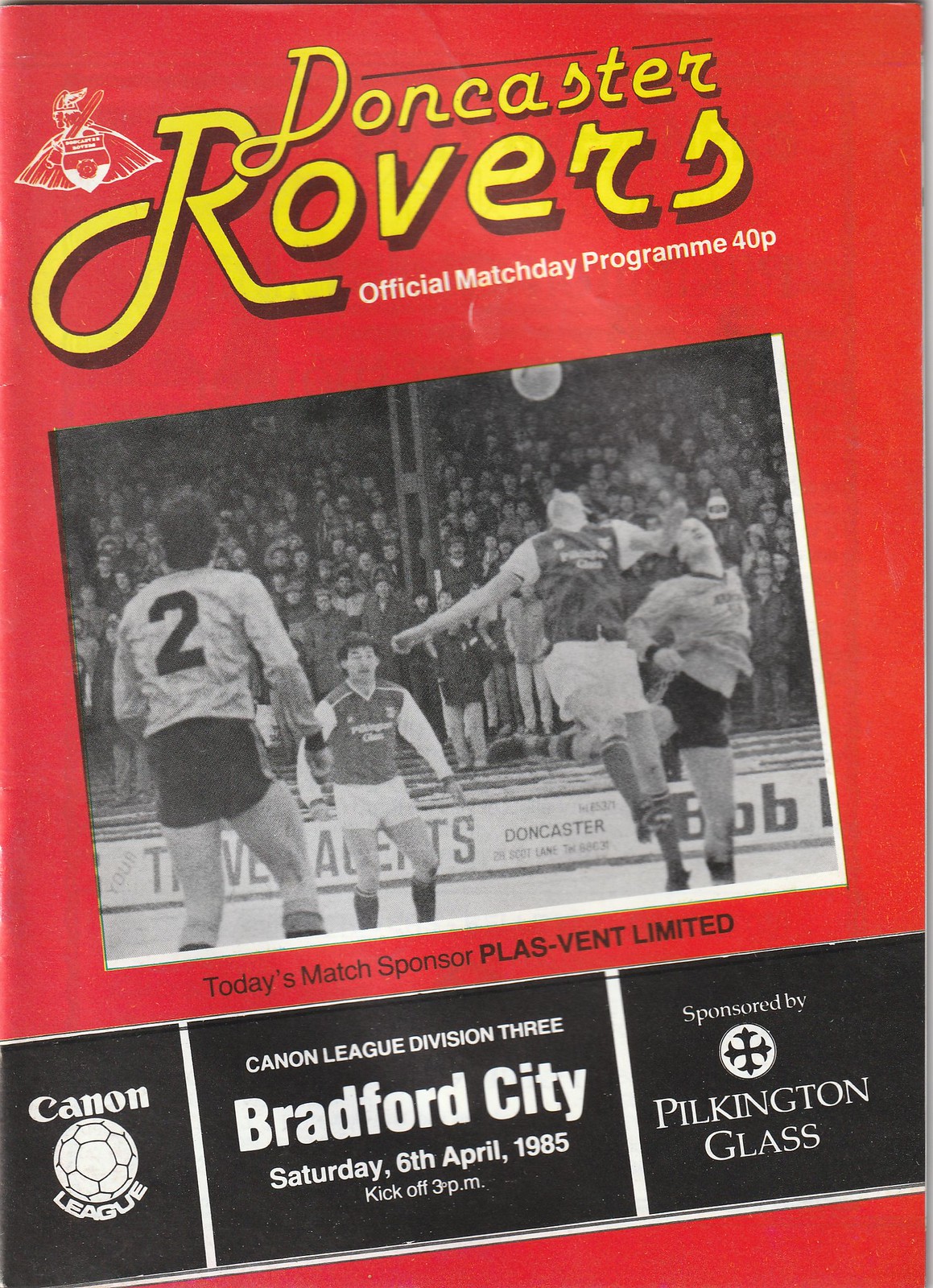This image is the cover of an old sports magazine, specifically an official match day program for a Doncaster Rovers game. The cover is a tall, rectangular shape with a bright red background. At the top, in a large, yellow, slightly cursive text that slants diagonally upwards to the right, it reads "Doncaster Rovers," with a team emblem to the left. Beneath this, in white letters, it states, "Official Match Day Program 40P."

Centrally located on the cover is a black-and-white photograph, slightly staggered diagonally, depicting an intense soccer match. The ball is airborne near the top right corner of the image, and four players are heavily involved in the action. Players wear distinct uniforms: one team in white shorts and gray/white shirts, and the other in white shirts with black shorts. The background is filled with spectators, all dressed in shorts, observing the match closely.

Below the photograph, a black bar runs parallel, displaying the text "Today's Match Sponsor, Plaz-Vent Ltd." Additionally, it includes details such as "Canon League Division 3," and mentions the match between Doncaster Rovers and Bradford City, scheduled for Saturday, 6 April 1985, with a kickoff at 3 p.m., sponsored by Pilkington Glass. This detailed cover serves not just as a match day guide but also a historical snapshot of the era's sports culture.